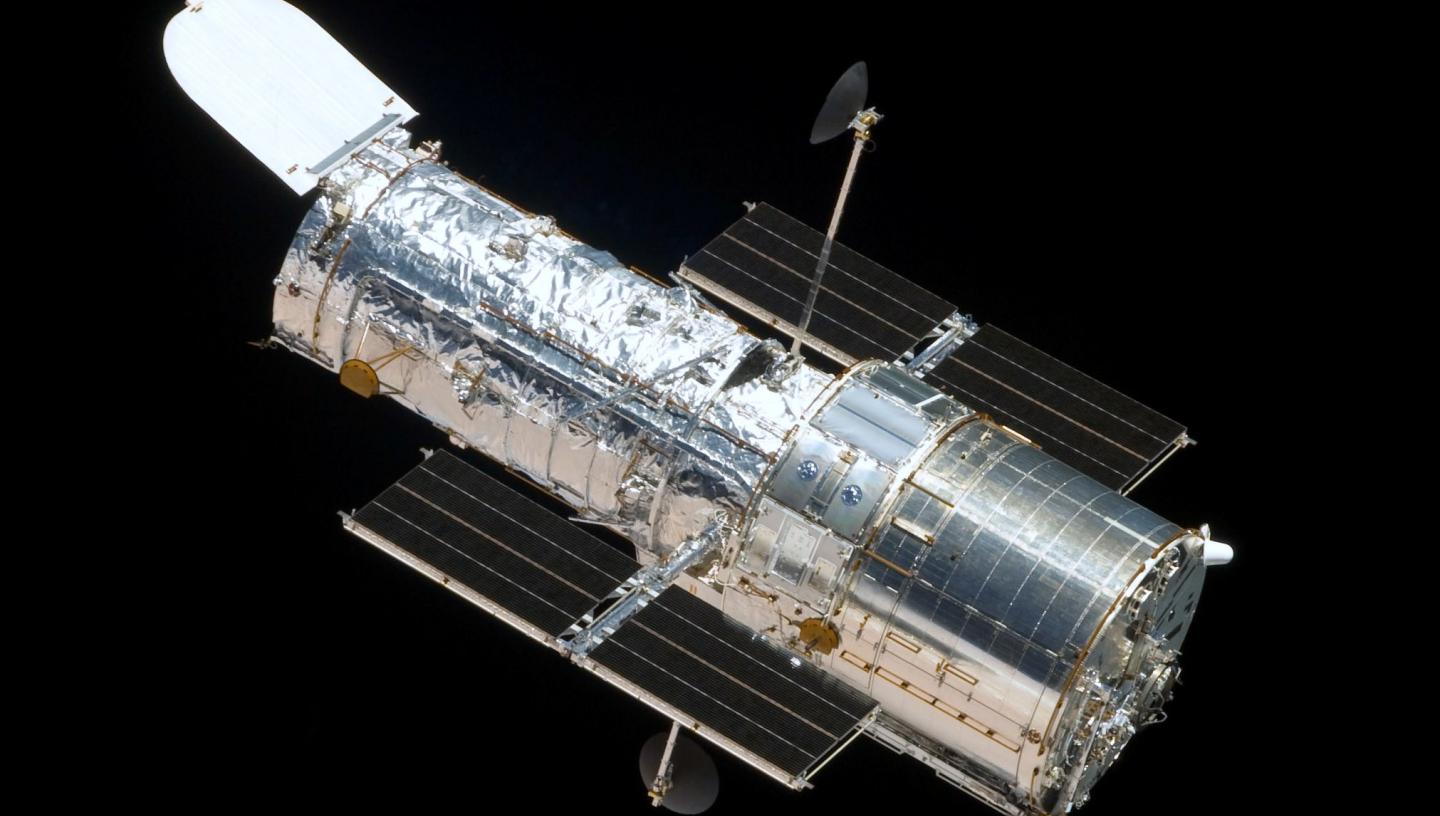The image depicts a detailed rendering of a spacecraft or satellite floating against a solid black background. The central structure is a crinkly, silver aluminum cylinder, resembling tinfoil. Extending from the cylinder are two solar panels, designed as long, horizontal black and white lines positioned on the near and far sides. A notable feature is the white hatch on the top left, open and reminiscent of a mailbox lid. Additionally, an antenna with a dish is mounted on a post stemming from the cylinder. Below this main body, the cylinder is connected to a metallic base resembling a silver paint can. The scene is devoid of text, maintaining a focus on the neutral color palette of black, white, gray, with subtle brown and yellow accents. Every element contributes to the lifelike depiction of a sophisticated space vehicle suspended in the void.